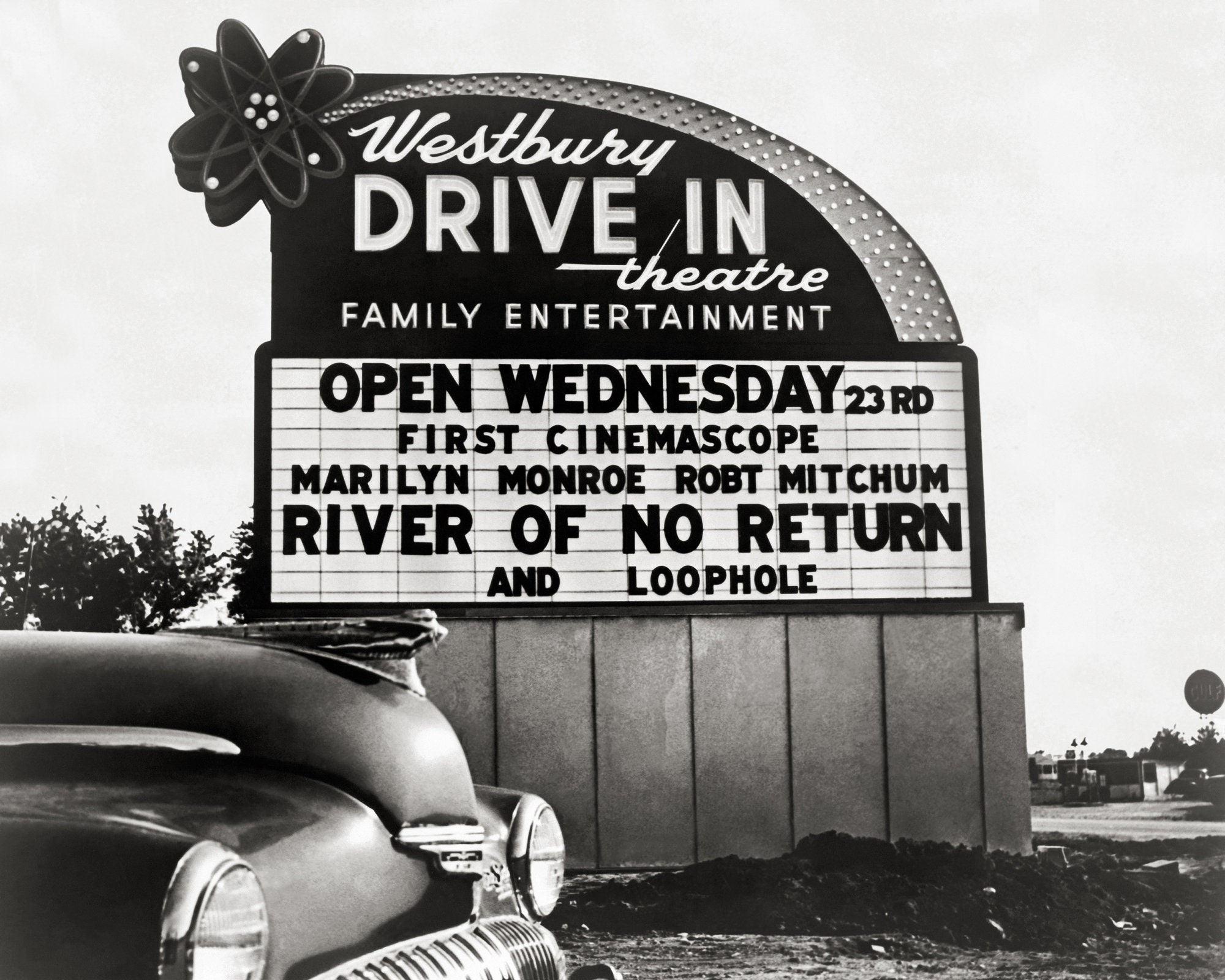This detailed black and white photograph captures an evocative scene from a bygone era, featuring the outside signage of the Westbury Drive-In Theater, set against a white sky typical of monochrome photography. The vantage point is from the ground level, providing a side view that includes an old-timey car in the bottom left corner. The car, light in color, prominently showcases its white-trimmed hood, with circular headlights encased in silver on each side. The partially visible front grill emerges slightly from below, while a large mound of dirt sits in the foreground.

The drive-in sign itself dominates the image, exuding a retro style characteristic of the 1950s or 60s. In the top right of the sign, a design resembling an atom with a silver line across its black background holds illuminated text reading, "Westbury Drive-In Theater Family Entertainment." Adjacent to this, the top left corner of the sign is adorned with a large, stylized flower.

Beneath this header, the marquee displays the message, "Open Wednesday, 23rd, First CinemaScope, Marilyn Monroe, Robert Mitchum, River of No Return, and Loophole," indicating a nostalgic film lineup. The sign is supported by a concrete wall, adding to its sturdy presence. Trees, a house, and a stop sign populate the background, framing the scene in an authentic snapshot of mid-20th century Americana. The photograph’s black and white aesthetic further enhances its vintage charm.